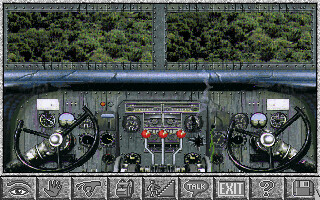The image appears to be a screenshot from a video game. It showcases a central structure that resembles a hybrid between a train and a large truck, featuring multiple wheels and gear-like mechanisms at its core. Surrounding this central vehicle, the scene includes various elements such as trees and a silver section that could represent a road or metallic surface. 

At the bottom of the screen, there is a user interface menu with several icons, each symbolizing different actions: a hand, a figure walking upstairs, a conversation bubble, an exit symbol, a question mark, and a CD icon, likely indicating a save option. This detailed layout suggests that the image is from a specific in-game menu, possibly a save or settings screen.